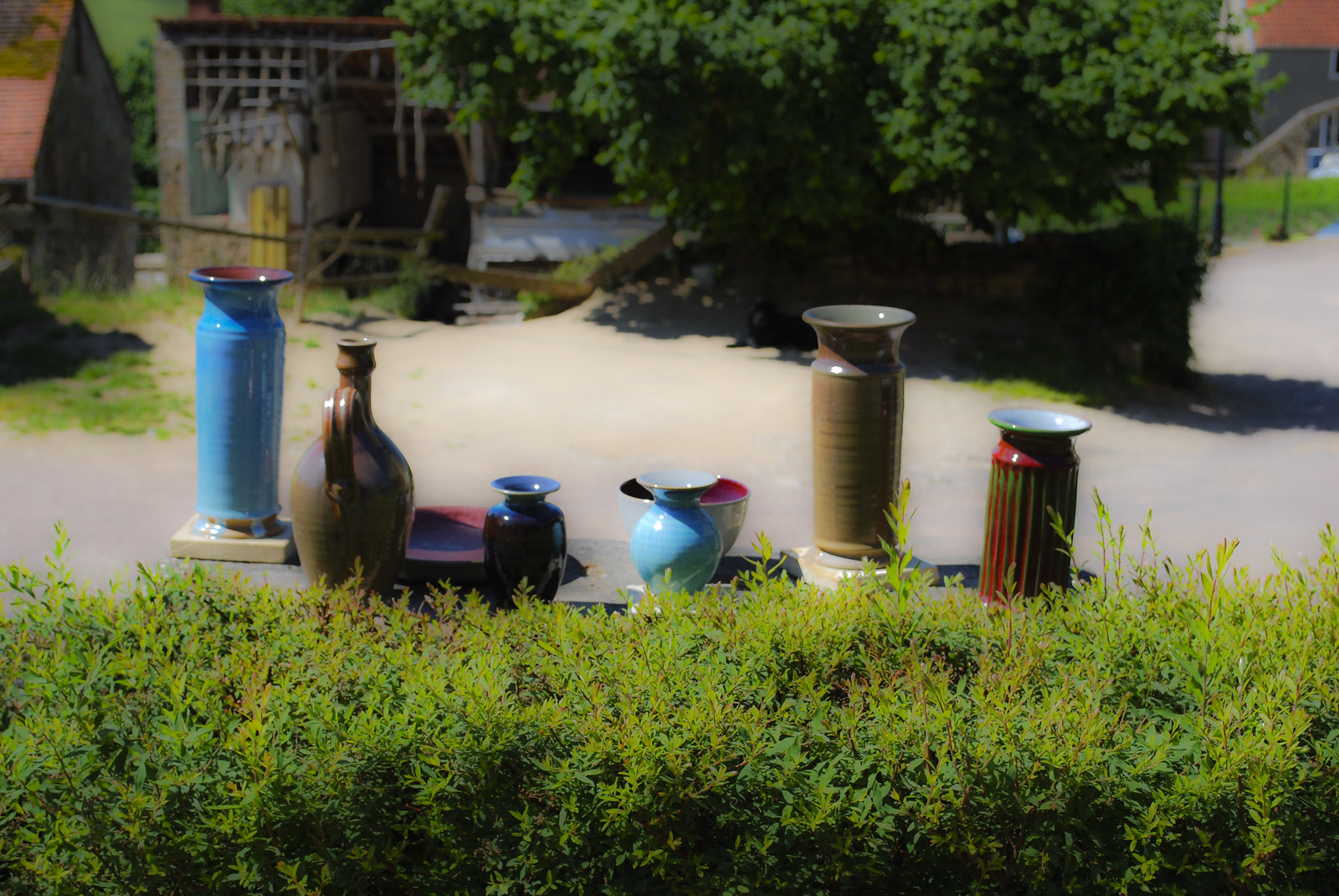The image captures an outdoor setting featuring a variety of decorative pottery positioned prominently in the foreground. Situated on a ledge, the collection includes six different pottery pieces alongside a bowl. From left to right, they are: a tall, light blue vase; a brown vase with a handle; a short black vase; a short blue vase; a tall, light brown vase; and a medium-sized vase that transitions from red to green. A bowl with a red trim on the inside is partially hidden behind one of the vases. The pottery, while primarily circular in shape, varies in size and color.

The background showcases a lush, green environment with a mixture of bushes and a small tree, both casting shadows that confirm the image was taken in well-lit daylight. The bushes display a striking lime green color, more pronounced at their tips. A dilapidated wooden structure is also visible, adding a rustic charm to the scene. Overall, the well-arranged and vividly colored pottery stands out against the verdant background, suggesting a decorative yet serene outdoor space.